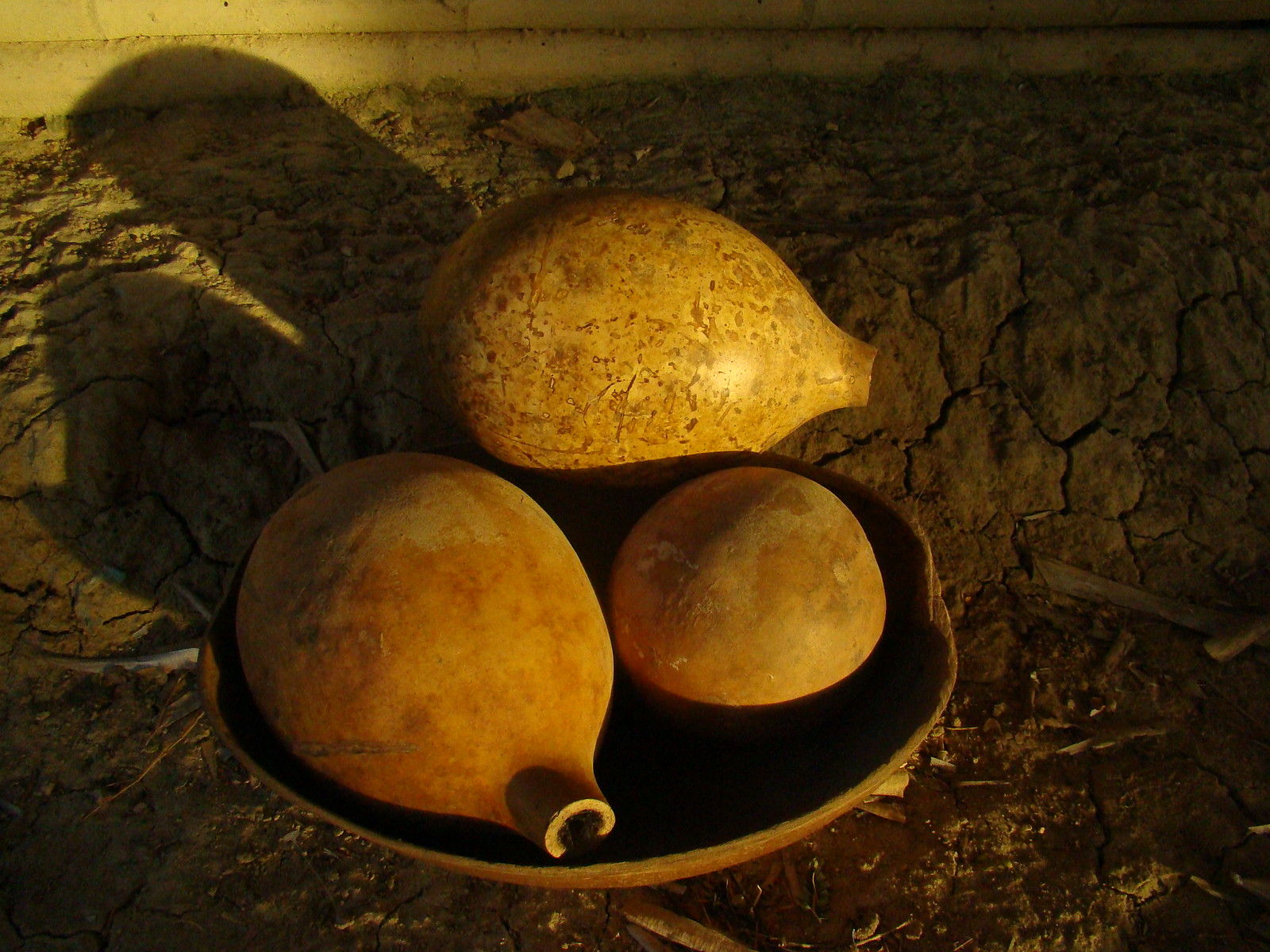In the image, there's a rocky, uneven ground covered with dry, hard dirt. This terrain appears rough and unlively. Dominating the foreground is an old, hand-carved container that might be made of metal or a flexible material. The container, resembling a pan or bowl, is central to the scene and looks ancient, potentially from tribal times. Inside this container, there are three gourd-like objects or very hard, pear-shaped fruits. These items are brownish, with one appearing yellow and showing signs of significant age, possibly hundreds of years old. The objects have a hardened, dinged exterior and seem hollow, with the tops cut off, suggesting they could have been used as drinking vessels. The setting is dimly lit, casting shadows over the objects and enhancing the historical and rugged atmosphere of the scene.